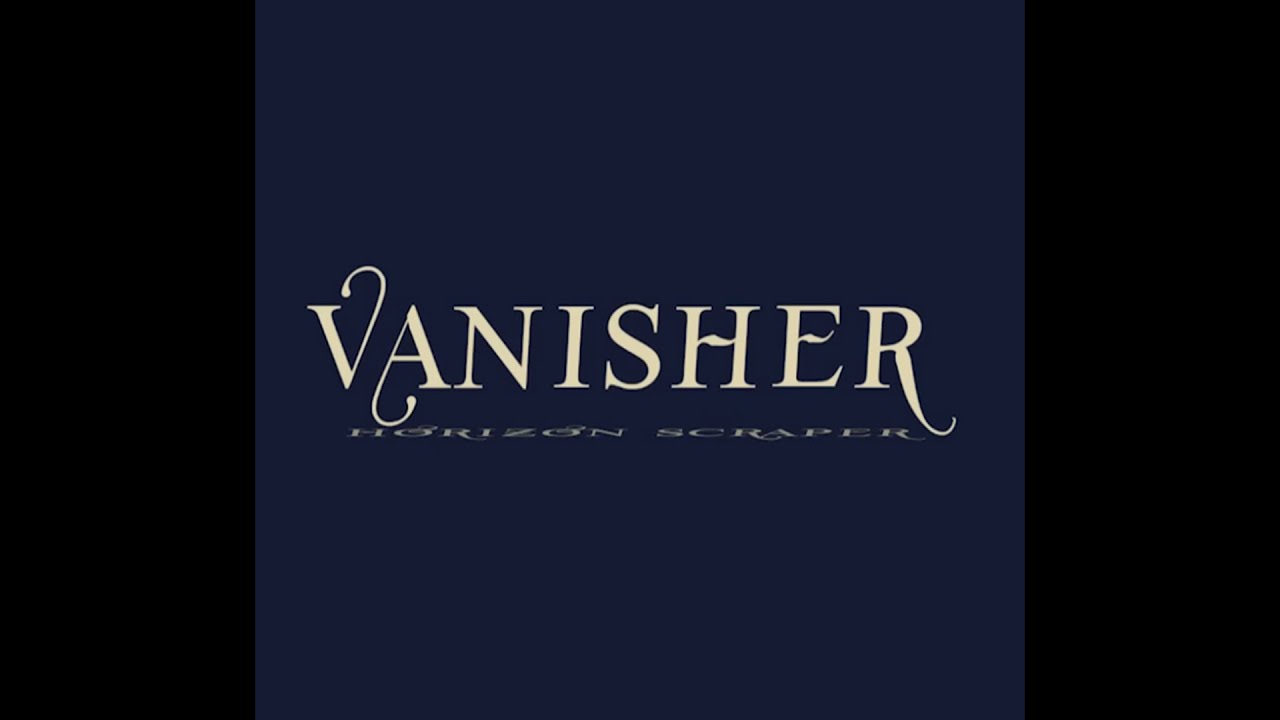The image is a 5 by 4-inch rectangular graphic with a solid dark navy background. At the center, in light cream or beige block letters, is the word "VANISHER" in all caps. The unique, standout feature of the lettering includes stylish hooks or curls: the right side of the "V" extends up in a hook shape, the left side of the "A" curls downwards like a "J," and the "R" has an extended leg that curls back up. Below "VANISHER," there is a compressed text that reads "HORIZON SCRAPER," though it is difficult to decipher due to the squished appearance of the lettering.